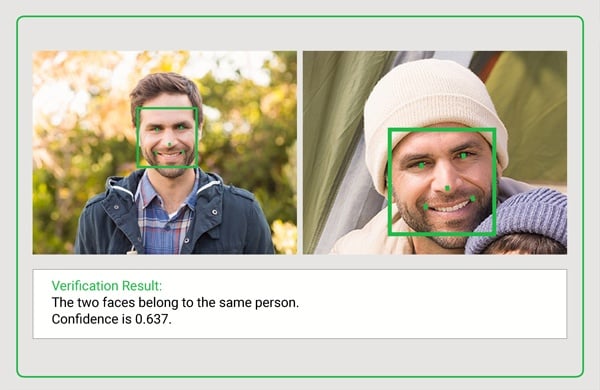The image shows a facial recognition verification result featuring two pictures of the same man. Both images are enclosed within a gray rectangular box bordered by a thin green line. The top left image presents a smiling man with brown hair and a beard, standing in front of a backdrop of vegetation featuring greens, browns, and whites. He is dressed in a blue jacket with white details, layered over a blue, red, and white checkered shirt. A green square highlights his face, pinpointed by five green dots positioned at his eyes, the tip of his nose, and the corners of his mouth. 

The image on the right depicts the same man wearing a white hat, possibly with a child in his lap. His face is similarly framed by a green square with corresponding green dots at the same facial landmarks. Below these images, in green text, is the phrase "Verification Result," followed by the statement "The two faces belong to the same person." The final line reads, "Confidence is 0.637."